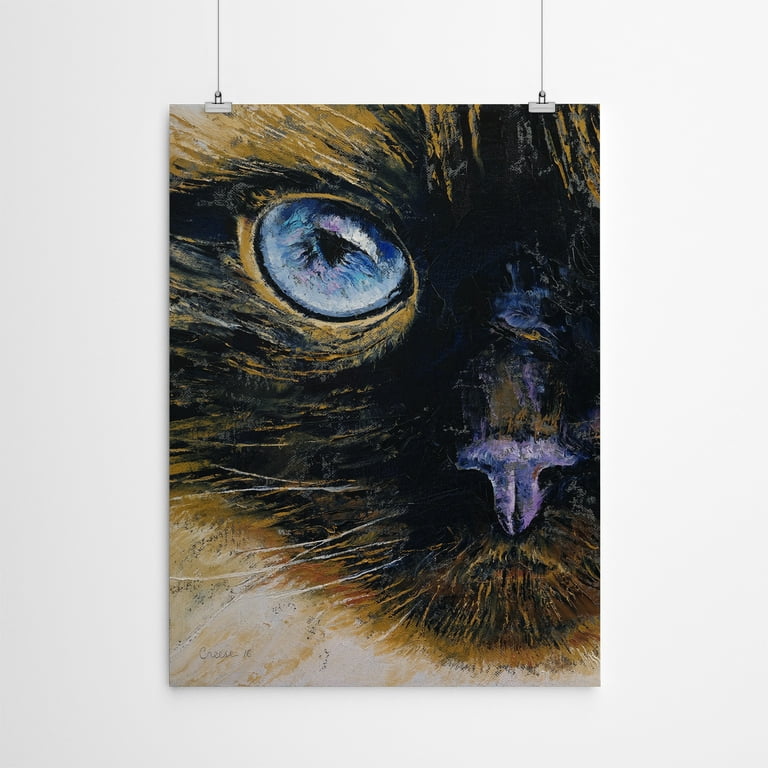This is a detailed painting of an extreme close-up of a cat's face, prominently featuring one eye and its nose. The focus is on the right side of the cat's face, capturing the intricate details of the fur, whiskers, and facial features. The cat's eye is a striking light blue with streaks of violet, set against its dark fur that fades into a brown hue around the eye. The nose, a darker bluish-violet shade, leads down to a barely visible mouth. The painting highlights the textures and patterns of the cat's fur and whiskers, with the white, wiry whiskers standing out against the dark backdrop of the face. The entire piece is displayed on a blank gray wall, hanging from two clips attached to strings at the top. The close-up perspective allows viewers to look directly into the cat’s eye, making the painting appear as though the cat is staring dead-on at the observer.